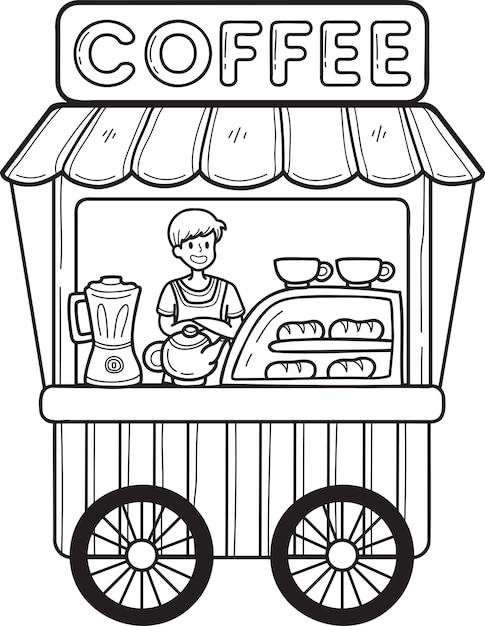This black-and-white drawing portrays a detailed line art image of a vintage-style coffee cart, suggesting a scene ready for coloring. The cart features two large black-spoked wheels supporting a rectangular base. At the top, a marquee-style sign with rounded corners prominently displays the word "COFFEE." The cart has an awning with striped, convex ends that curve downward, giving it a nostalgic look. 

Behind the counter stands a person with short hair, wearing a t-shirt and an apron. The counter is adorned with various items: on the left, there is a blender; in the middle, a teapot; and to the right, there's a glass-encased display case containing four loaves of bread arranged in two tiers. On top of this display case sit two teacups. The image captures a quiet moment at the coffee cart, emphasizing the preparation area and its inviting setup.